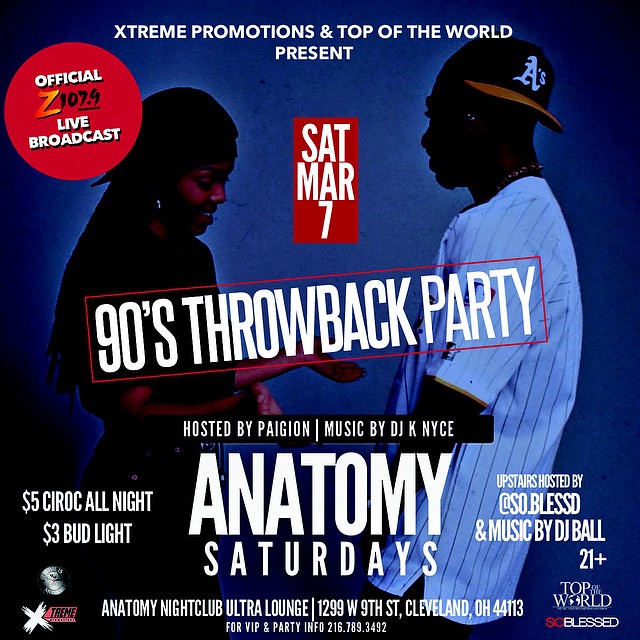The promotional image for the "90's Throwback Party" is vibrant with blue, white, and red colors, hosted by Extreme Promotions and Top of the World. At the top in bold white letters, it's announced as an official live broadcast on Z107.9, taking place on Saturday, March 7th. The hosts for the evening are Page Ian and DJ K Nice, with additional entertainment by DJ Bo and It's So Blessed.

The background features a black woman on the left and a black man on the right, both dressed in 90s-style attire. The woman wears a backwards black baseball cap with long braided hair and extends her arm as if shaking hands. The man sports a white striped baseball jersey and a backwards cap with the A's logo. 

Information about the venue is displayed prominently: the Anatomy Nightclub Ultra Lounge, located at 1299 West 9th Street, Cleveland, Ohio, 44113. The event is 21 and over, featuring drink specials including $5 Ciroc all night and $3 Bud Light. 

For VIP and party info, attendees are encouraged to contact 216-789-3492. Extreme Promotions' logo is placed in the lower left corner of the image, while other details about the event are scattered across the design.